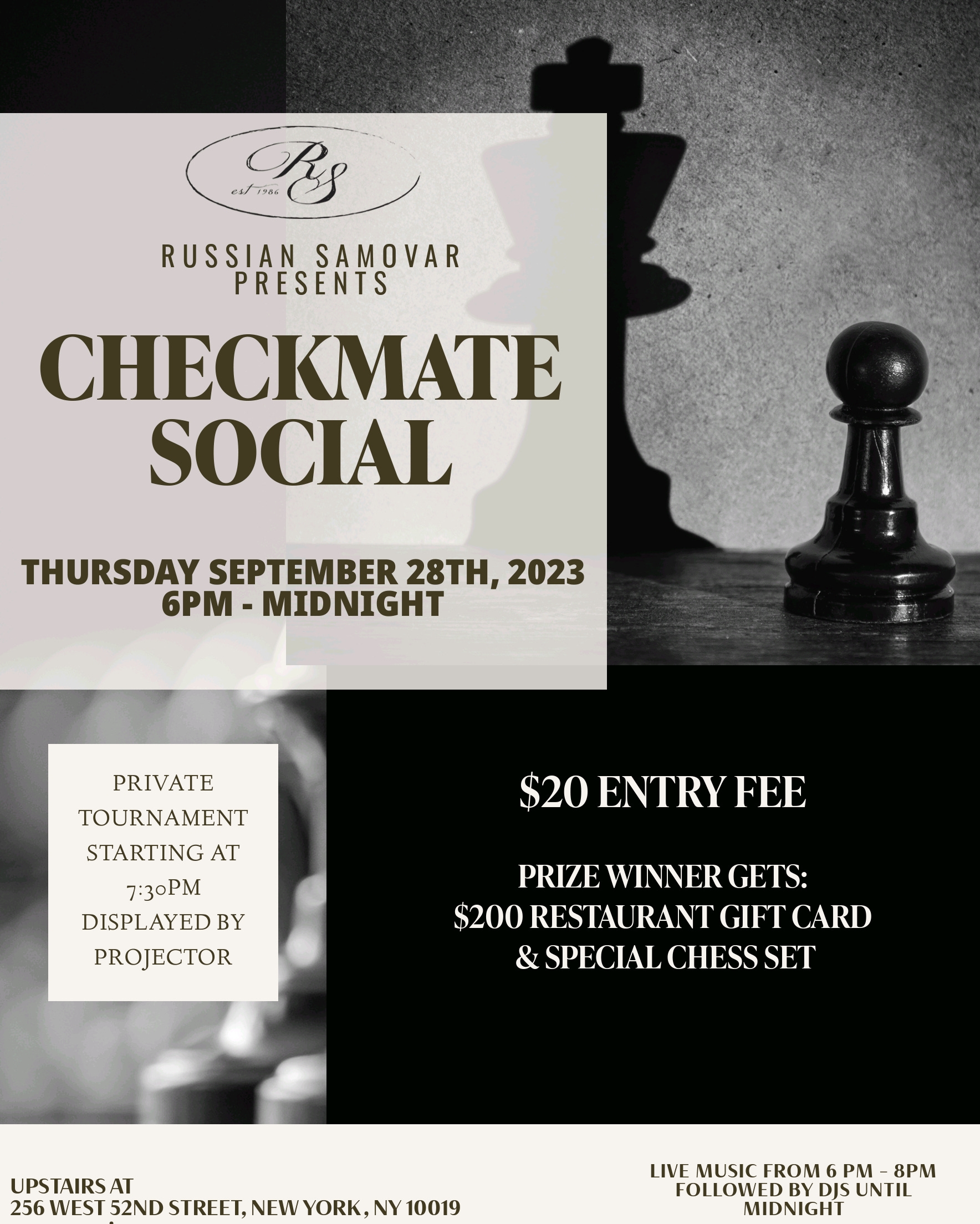This promotional poster advertises an event titled "Checkmate Social" hosted by Russian Samovar. Dominated by a monochromatic theme, the background features chess pieces set on a dark surface with a gray wall backdrop. On the left side, a prominent white square contains black text that reads "Russian Samovar Presents" above the logo with the initials "RS". Just below this, it says "Checkmate Social" in large black letters followed by the details "Thursday, September 28, 2023, 6 p.m. to midnight". 

Towards the right, white text against the dark background informs attendees of a "$20 entry fee" and that the "prize winner gets a $200 restaurant gift card and a special chess set". Additionally, the poster highlights a private tournament starting at 7:30 p.m., with the event featuring live music from 6 to 8 p.m. followed by DJs until midnight. 

Two images are also featured: a black and white photograph on the top right of a chess pawn casting the shadow of a king, and a blurry, out-of-focus photograph of white chess pieces at the bottom left. The bottom part of the poster adds a final note in green text: "Upstairs at 256 West 52nd Street, New York, NY 10019", indicating the event location.